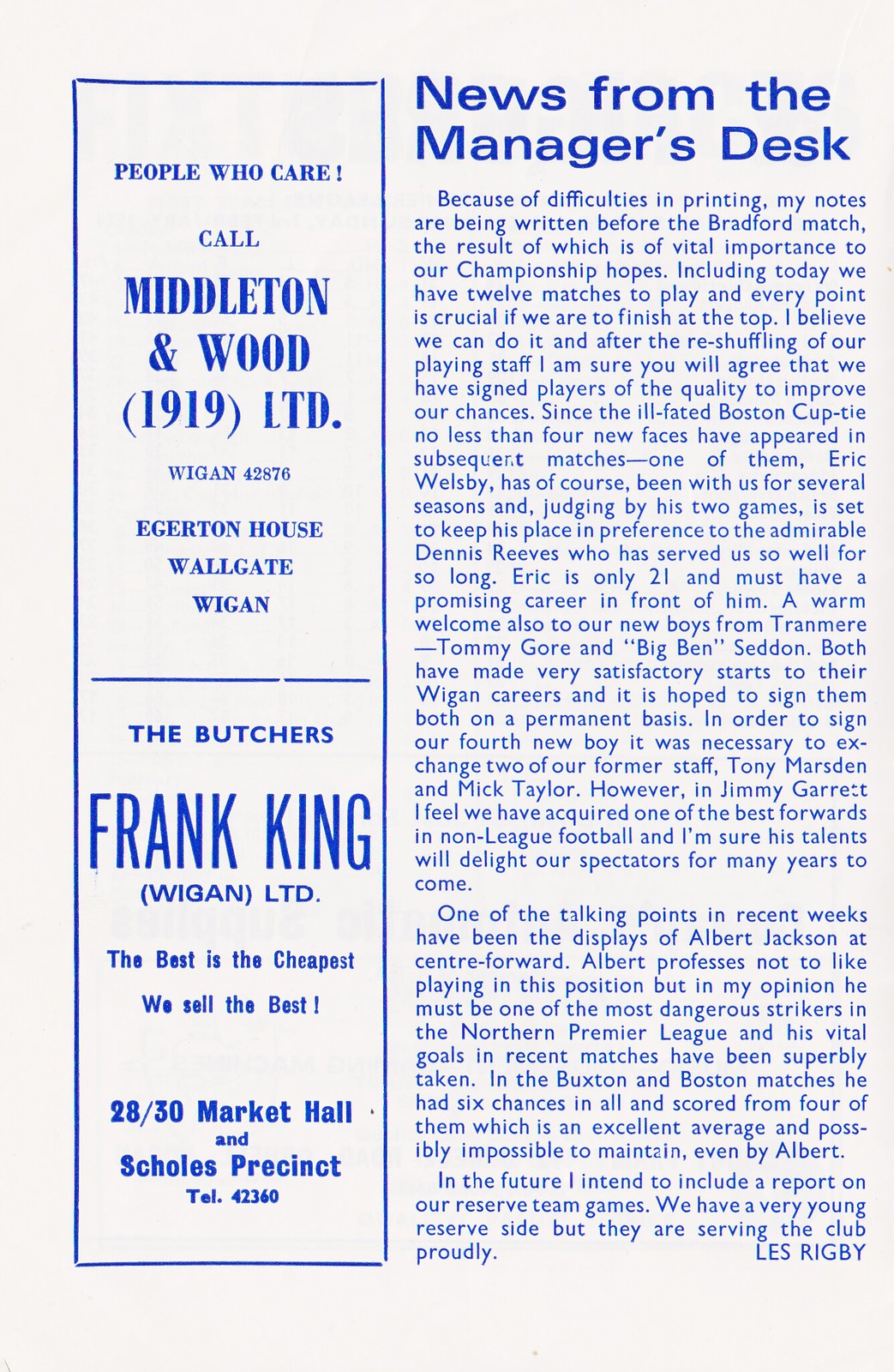The image appears to be an excerpt from a vintage article with a white page background and entirely blue-colored text. On the left side, there are two vertical boxes with blue borders, stacked on top of each other. The top box reads, "People Who Care, Call Middleton and Wood, 1919 Limited, Wagon 4 to 8 7 6, Egerton House, Ballgate, Wigan." The bottom box contains an advertisement for a butcher: "The Butchers, Frank King, Wigan Limited. The best is the cheapest. We sell the best. 28 30 Market Hall, Schools Present. Tel: 4 2 3 6 0."

On the right side, the article is titled, "News from the Manager's Desk." The content discusses the manager's notes before an important match against Bradford, emphasizing the importance of winning to maintain championship hopes. The manager notes the addition of four new players, including Eric Willsby, who is expected to take a prominent role, and recent signings from Tranmere, Tommy Gore and Ben Seddon. The article also highlights the performance of Albert Jackson at center forward, praising his goal-scoring capabilities. The commentary concludes with a mention of the reserve team, stressing the promise and dedication of the young players. The article ends with the signature, "Less Rigby."